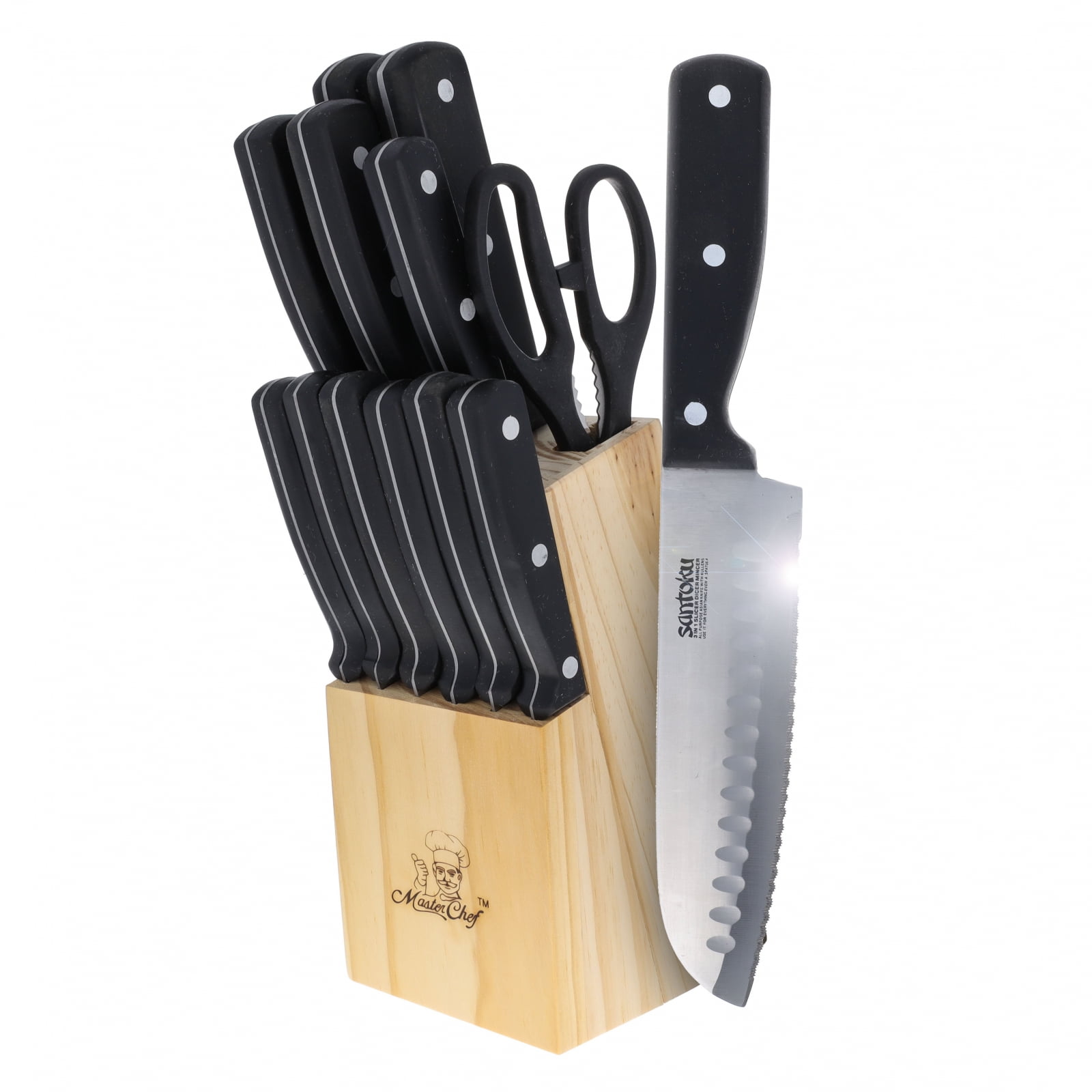This image showcases a comprehensive MasterChef™ Santoku knife set, featuring a wooden butcher's block with dedicated slots for each knife. The set includes six steak knives, a pair of scissors, and a variety of other knives, including a serrated knife, though some specific knife types are not clearly identified. The knives feature black plastic handles adorned with silver screws. Notably, the knife block bears the MasterChef™ branding, and one knife, with a shiny blade reflecting camera light, has been pulled out. Positioned against a crisp white background, the detailed components and the striking sheen of the knife blade make the set aesthetically appealing and functional for various culinary tasks.